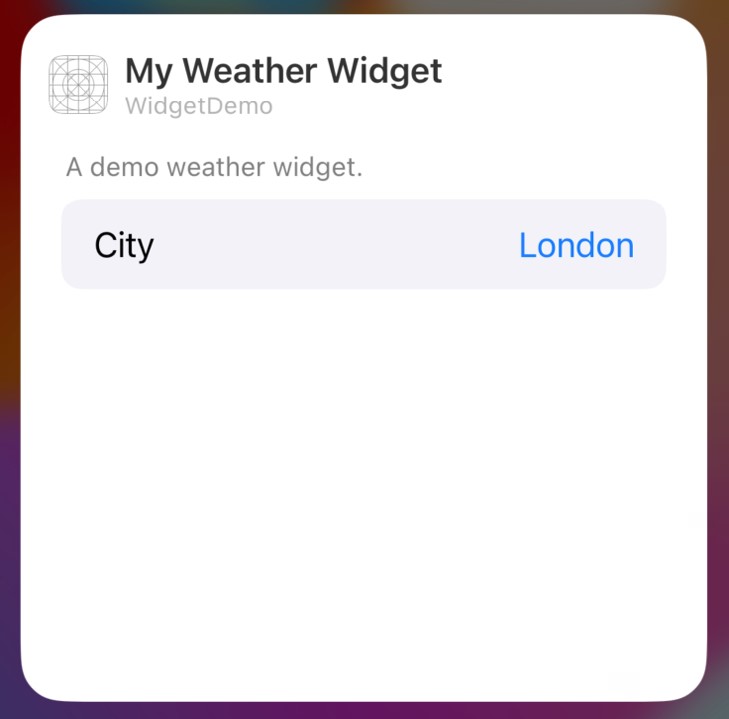This image features the settings screen of a weather widget displayed on an iPad or iPhone, identifiable by the distinctive system font. The central dialogue box is bordered by a mosaic of muted colors: reddish, greenish, bluish, purplish, and brownish hues that blend randomly without discernible patterns or images, suggesting a blurred or abstract background.

The dialogue box has a clean design with black text on a white background. At the top, the widget is titled "My Weather Widget." Just below, there is a lighter gray subheading, "Widget Demo." Further down, in smaller black text, the description reads "Demo Weather Widget."

At the bottom of the dialogue box, there is a gray rectangular area, which appears to function as a settings field for user preferences. Inside this area, on the left, is the label "City" in black text. On the right-hand side, the word "London" is displayed in blue text, indicating the current selected city for the weather widget.